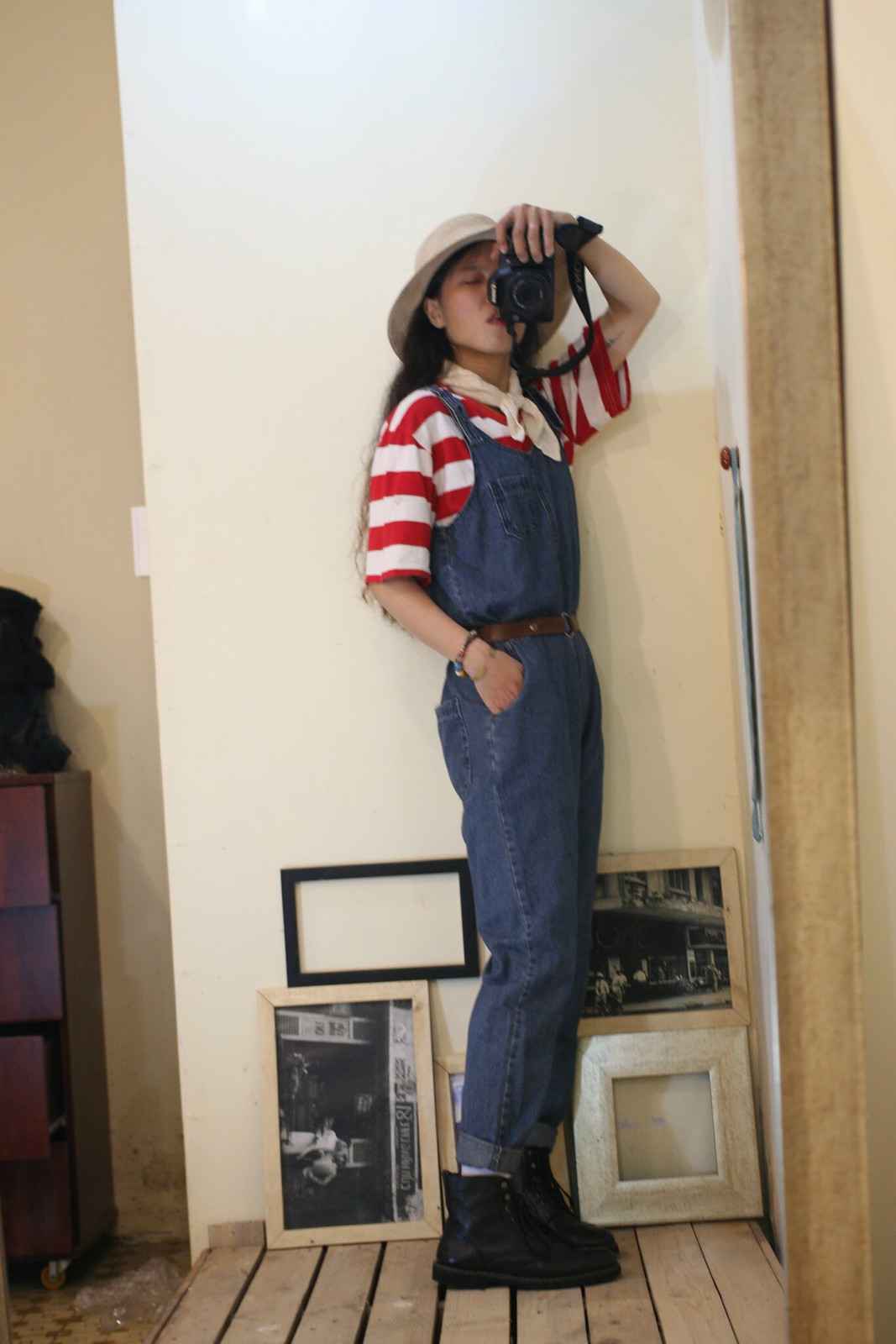This vibrant color photograph captures a young Asian woman standing sideways on a light-colored wooden plank surface, with an assortment of picture frames stacked behind her legs. She has long, straight black hair that falls to the middle of her back and is partially obscured by a white brimmed straw hat. Dressed in denim overalls cinched at the waist with a brown belt over a short-sleeved red and white striped shirt, she exudes a casual yet stylish vibe. The woman's right hand is tucked into her pocket, while her left hand is raised, holding a black DSLR camera with a strap hanging down around her wrist, covering half of her face as she appears to be taking a selfie, possibly in a mirror. Behind her, there are five wooden frames of varying colors; three contain black and white photos, while two are empty. Her eyes are almost closed, adding a serene quality to the image. She completes her outfit with black boots and a white bandana tied around her neck, adding a touch of uniqueness and flair.